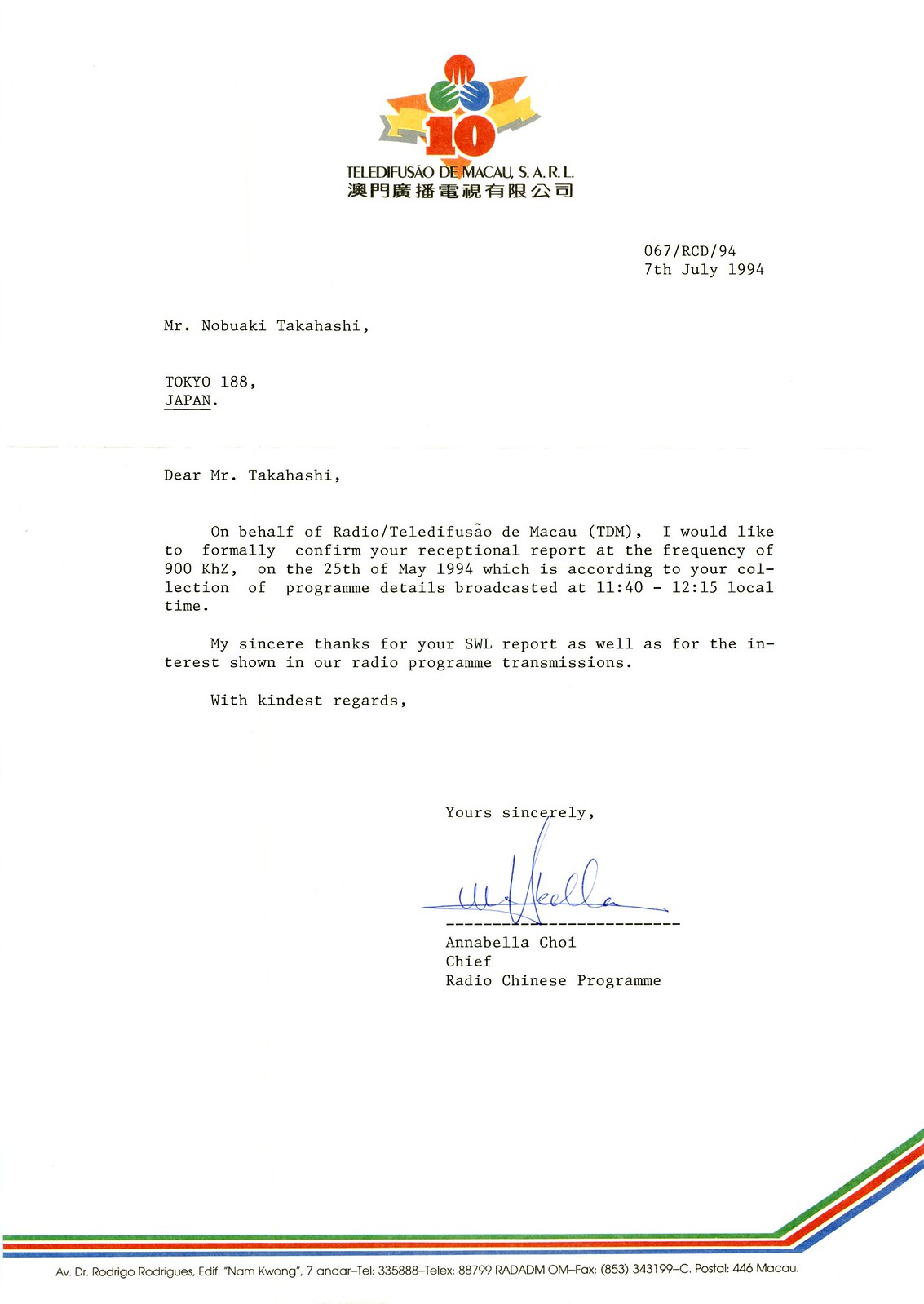This image captures a meticulously scanned or photocopied formal letter dated July 7, 1994, emanating from Telefusao de Macau, S-A-R-L, as indicated by its prominent letterhead and distinctive logo. The logo features an orange triangle encircled by a yellow ribbon, a large red "10" centrally placed, and a three-sided, fidget spinner-like emblem with red, green, and blue segments. The letter is addressed to Mr. Nobuaki Takahashi in Tokyo, Japan, and pertains to the confirmation of his reception report at the frequency of 900 kHz on May 25, 1994, based on his detailed account of program transmissions from 1140 to 1215 local time. The correspondence expresses gratitude for Mr. Takahashi's shortwave listening (SWL) report and his interest in their radio program transmissions, and it is signed by Annabelle Choi, the Chief of the Radio Chinese Program, concluding with "yours sincerely."